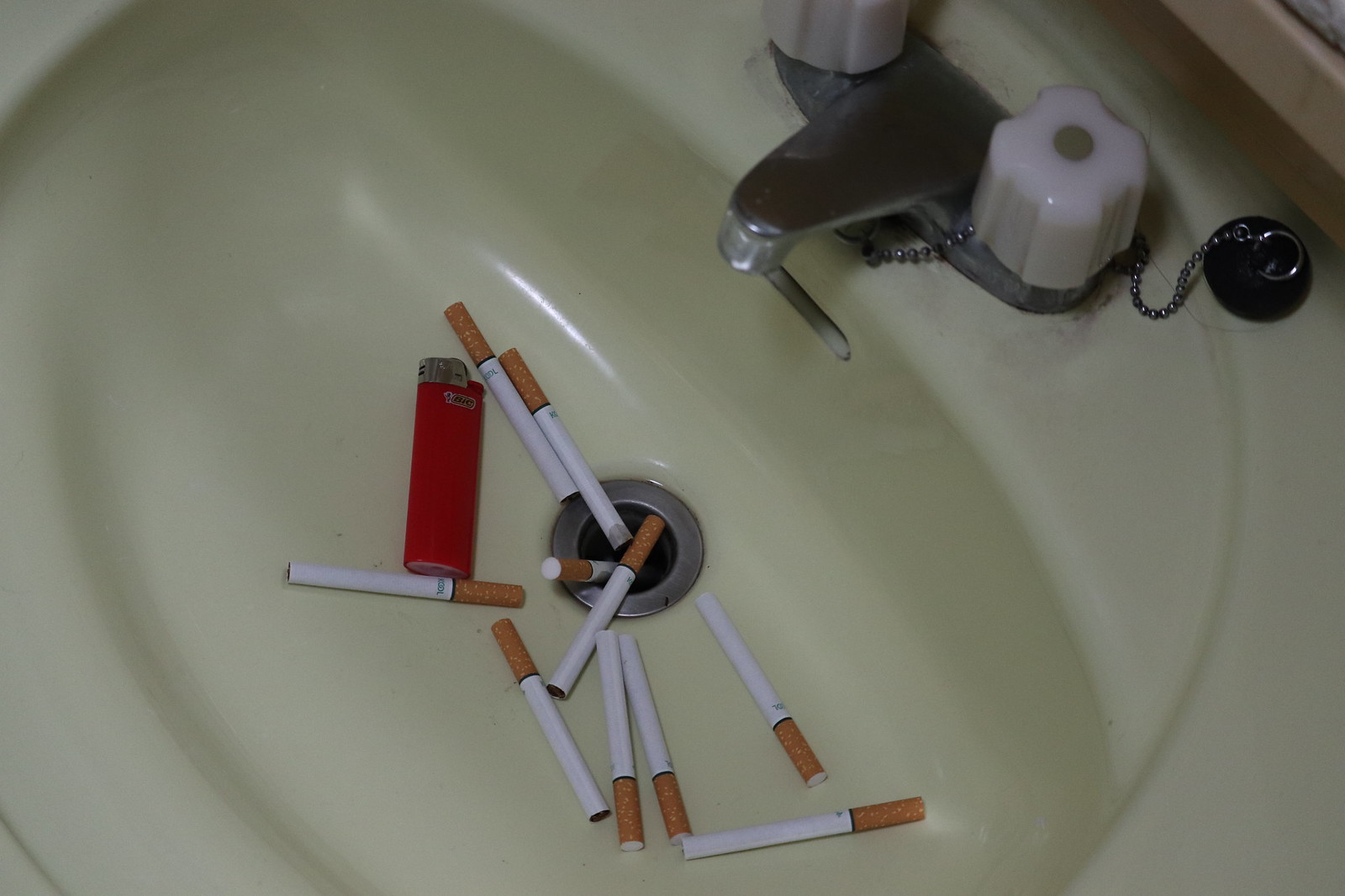This photograph depicts a slightly old-fashioned beige porcelain sink with a stainless steel faucet and white hot and cold water handles. The faucet is connected to a black drain plug on a silver chain. Inside the sink, there is a total of 10 cigarettes, each with white paper and cork-colored filters. Some cigarettes are scattered around the edge of the stainless steel drain, with three of them partially falling into it. To the left of the cigarettes, a red Bic lighter with a silver top rests prominently in front of the drain. The image is zoomed-in, focusing entirely on the basin of the sink and the objects within it.